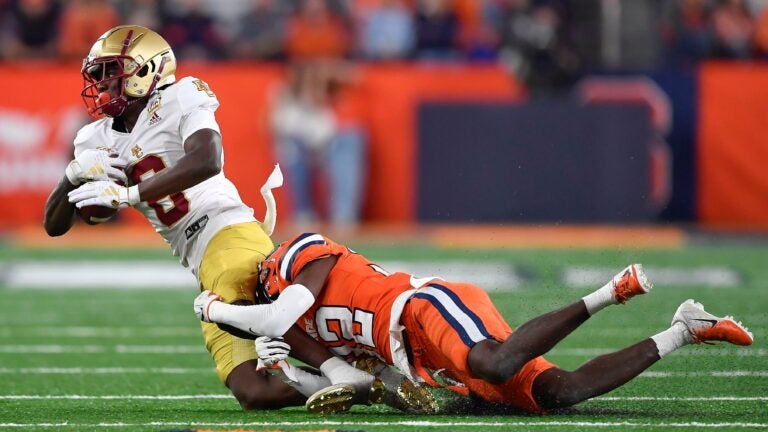In this dynamic and intense photograph, two African American football players are captured in action on a football field. The player in the midst of being tackled is wearing a gold helmet adorned with a maroon stripe, a white jersey displaying the maroon number 8, and yellow pants. He is in possession of the football and is in the process of falling to the turf. The tackler, who has grasped the ball carrier around the legs from behind, is dressed in a fully orange uniform with distinct black and white striping on both his sleeves and shorts. His uniform features the number 22, and he is wearing white socks along with orange and tan Nike shoes embellished with a black swoosh. The background is an out-of-focus blur of orange, suggesting the action takes place in an orange-themed stadium, likely that of either Syracuse or Clemson. The green astroturf field is clearly visible at the bottom of the image. The number 22 tackler's determined grip on the number 8 player illustrates the precise moment of defensive effort in football.